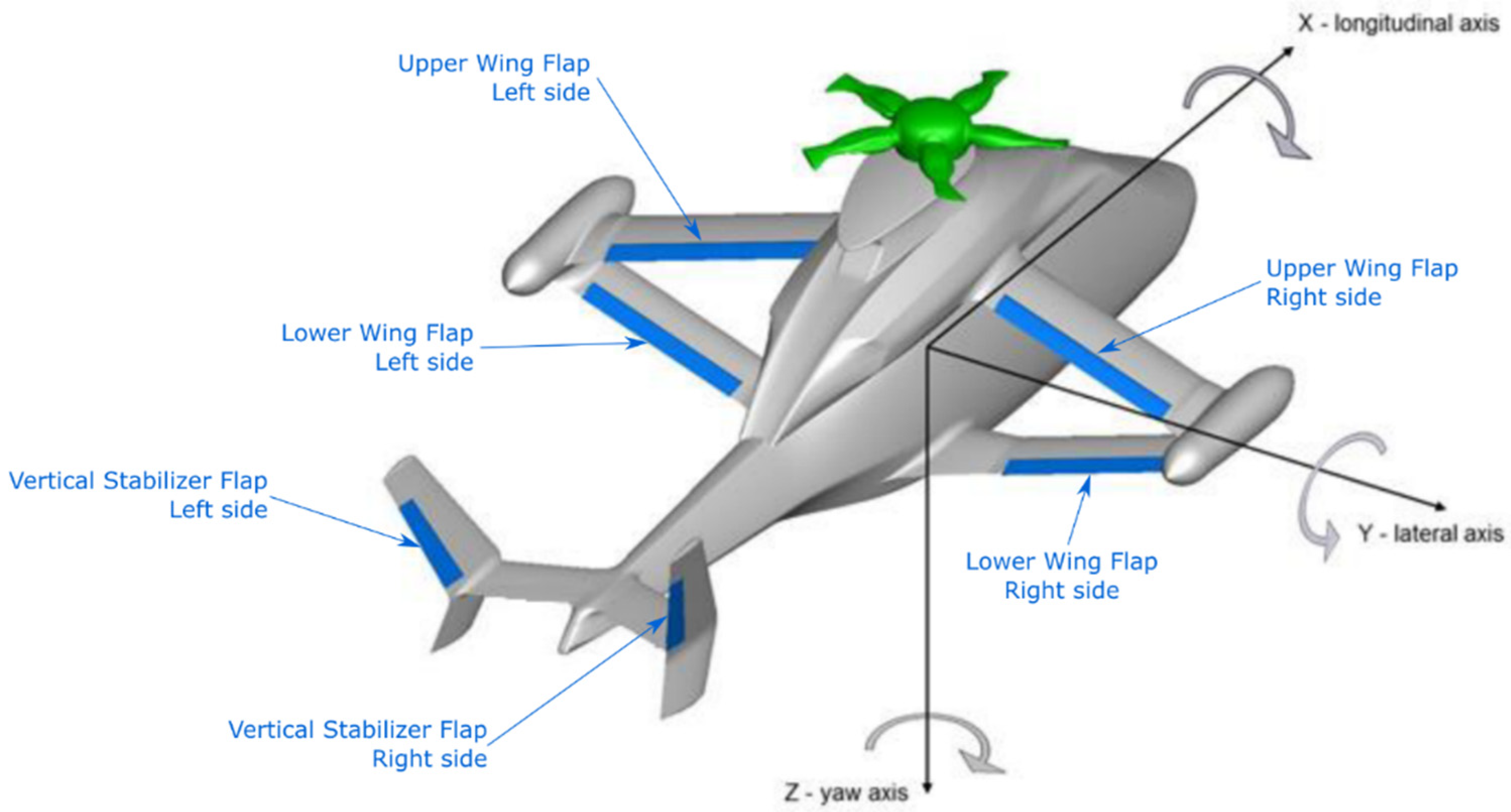The image is a detailed, computer-generated illustration of a helicopter. The helicopter features a gray body with blue lines along each side and the tail, creating a triangular pattern. It is shown from a slightly top-down perspective, with the tail pointing towards the lower left and the nose towards the upper right. At the top of the helicopter is a prominent, bright green rotor. The image includes numerous blue arrows pointing to different parts of the helicopter, such as the upper and lower wing flaps on both the left and right sides, and the vertical stabilizer flaps on both sides. Additionally, a large black arrow highlights the X longitudinal axis, Y lateral axis, and Z yaw axis. The illustration also shows a contraption that might be used for landing on water, and the helicopter has distinguishing blue stripes along its structure.